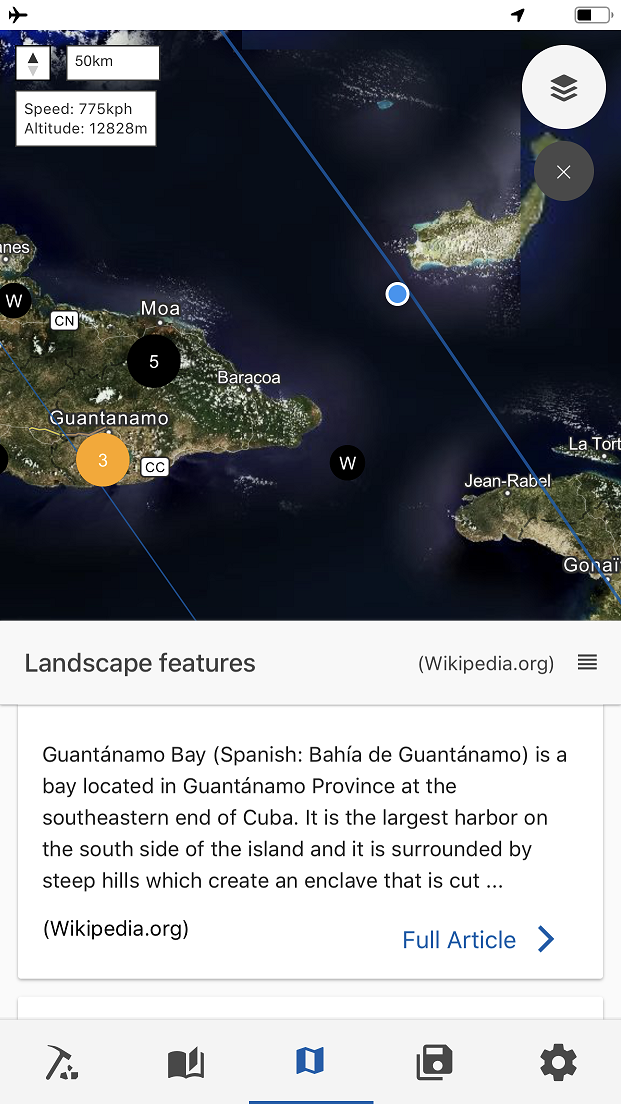This detailed image, sourced from Wikipedia.org, appears to be a screenshot taken from a mobile or tablet device currently in airplane mode, as indicated by the airplane icon in the upper left corner. 

In the upper right, navigation and battery icons are visible, showing the device's battery is slightly below halfway. The main focus of the image is a map prominently displaying Guantanamo Bay. Surrounding annotations include a yellow circle with the number "3" beneath Guantanamo, and a black circle with "5" located above the label "MOA." To the right of this is the town of Baracoa. A blue dot, typically representing the current location, is situated in the middle of the ocean near an unnamed smaller island.

The map features dark blue waters surrounding several islands, one of which is situated in the bottom right corner but remains unnamed. The map also includes info boxes displaying data such as speed and altitude. In the upper right corner of the map, there is a filter selection icon (a white circle with three black stacked squares) and a gray circle with a white "X" likely for closing the map.

Below the map, the image includes a label "Landscape Features," followed by "wikipedia.org" in parentheses. There's a hamburger menu icon offering a brief overview of Guantanamo Bay with an option to read the full article via a blue "Full Article" link accompanied by a right-pointing arrow. Additional icons below this section include a floppy disk symbol for saving and a gear symbol for settings, among others that remain unidentified.